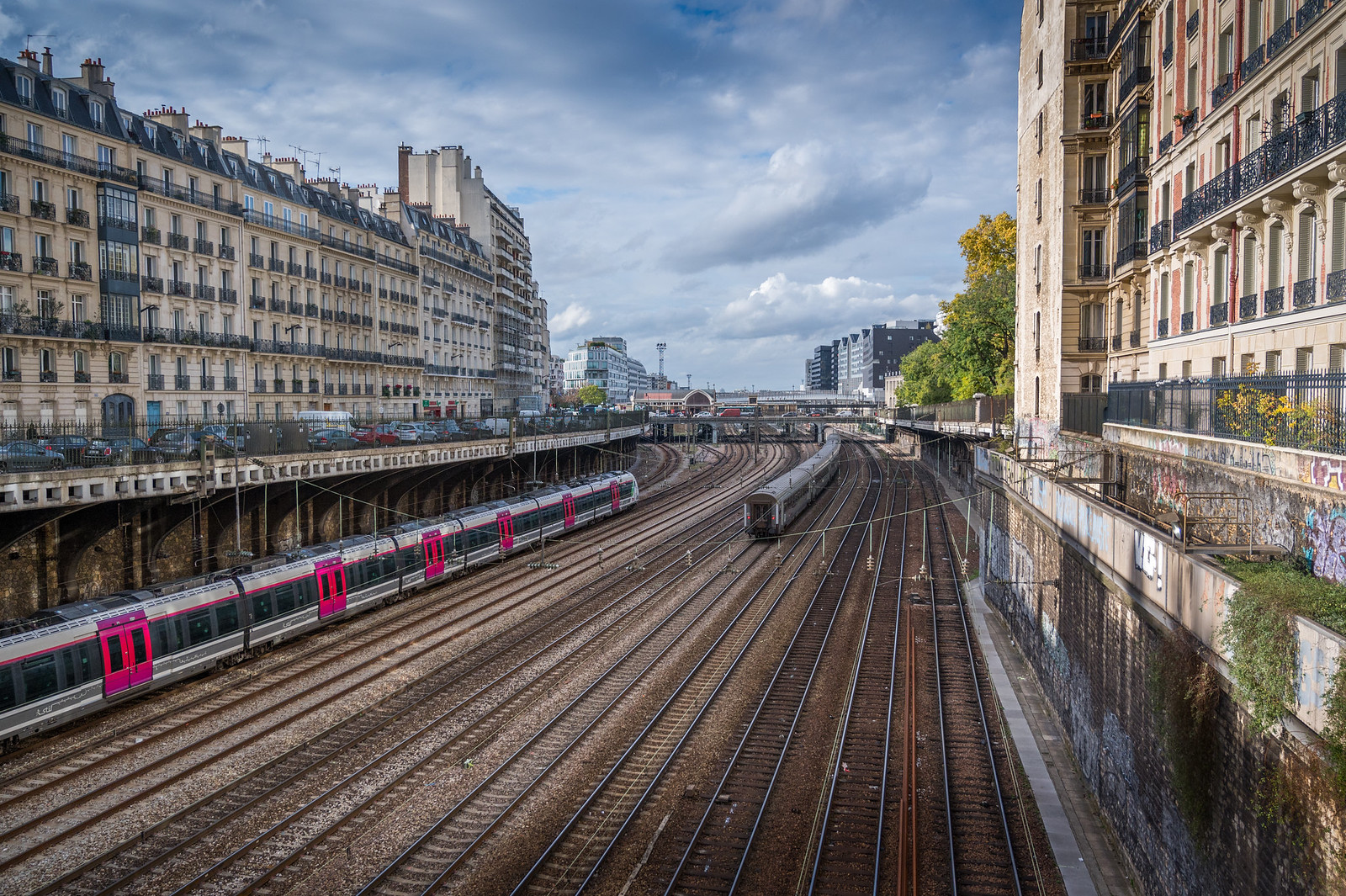The photograph presents a sweeping view of a large rail system flanked by two rows of buildings. There are more than ten parallel train tracks visible, cutting through the urban landscape. On the far left track, a train with a sleek silver and gray exterior and doors painted in deep pink is in motion. Another train is seen on the sixth track from the right, bearing a uniform gray steel-colored body.

To the left of the rail system, the buildings rise to six stories high, each adorned with chimneys, windows, patios, and balconies. These structures are elevated above the railway tracks, adding a sense of grandeur. Cars are intermittently parked along the street-level sections of the buildings.

Above, the scene is capped by a picturesque blue sky dotted with fluffy clouds, enhancing the overall charm of the urban setting.